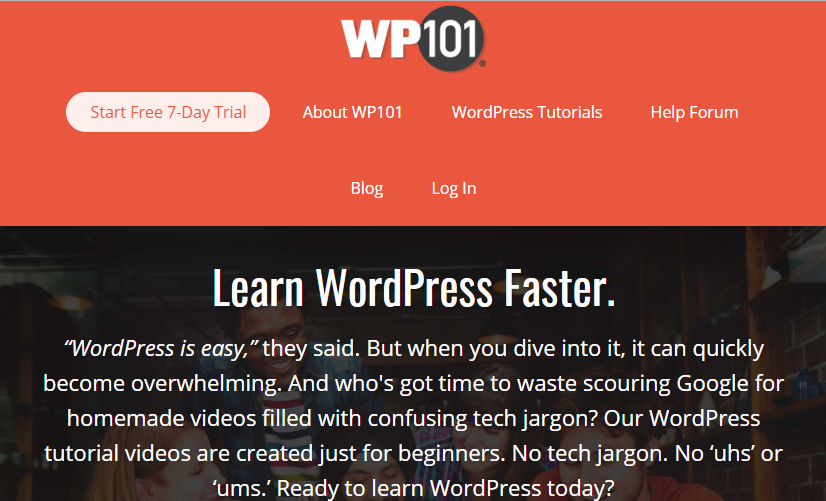This is a detailed and cleaned-up caption for the image:

---

The image is a screenshot from a WordPress website page, characterized by a vibrant reddish-orange header that spans the upper part. In the center of this header, the bold text "WP 101" is prominently displayed, with "WP" in capital letters and "101" enclosed within a black circle.

Below the header, the content is organized into clear sections. On the left side, there are several navigational options: "Start Free 7-Day Trial", "About WP 101", "WordPress Tutorials", and "Help Forum". Adjacent to these options, in the middle row, the page displays two succinct links: "Blog" and "Log In".

As you scroll down further, a prominent headline states, "Learn WordPress Faster", followed by a quote in smaller print that reads: "WordPress is easy, they said. But when you dive into it, it can quickly become overwhelming. And who's got time to waste scouring Google for homemade videos filled with confusing tech jargon? Our WordPress tutorial videos are created just for beginners. No tech jargon, no uhs or ums. Ready to learn WordPress today."

This comprehensive page layout is designed to cater to beginners, providing straightforward and jargon-free tutorials to ease the learning curve associated with WordPress.

---